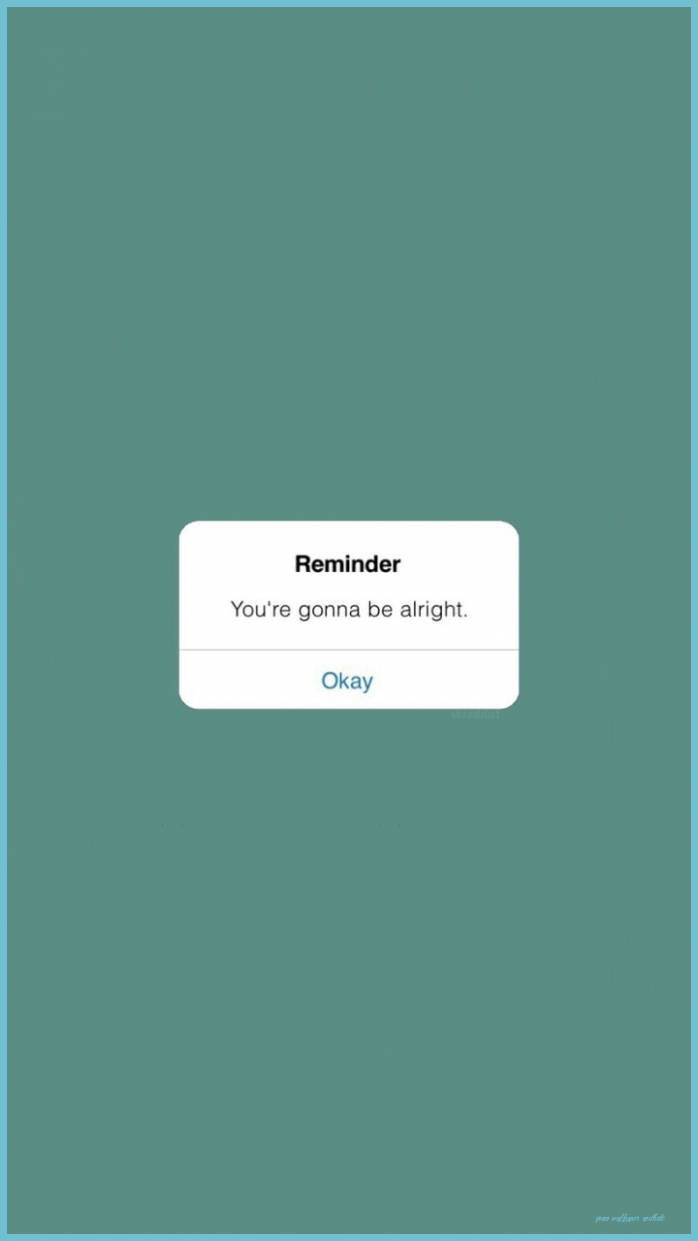The image appears to be a motivational notification, possibly from a wellness or mental health app designed for mobile devices or websites. The background features a calming greenish-teal color. The notification is displayed in a portrait-oriented rectangular box, approximately twice as tall as it is wide. Centrally positioned within this box is a smaller, white, rounded rectangle. At the top of this white box, in bold, black, centered text, is the word "REMINDER." Below it, regular black text reassures the viewer with the message, "You're gonna be alright." A faint horizontal line separates this text from the interaction option beneath it. In blue-teal text, the word "Okay" is displayed, likely functioning as a button to dismiss the notification. The overall design exudes a sense of reassurance and simplicity.